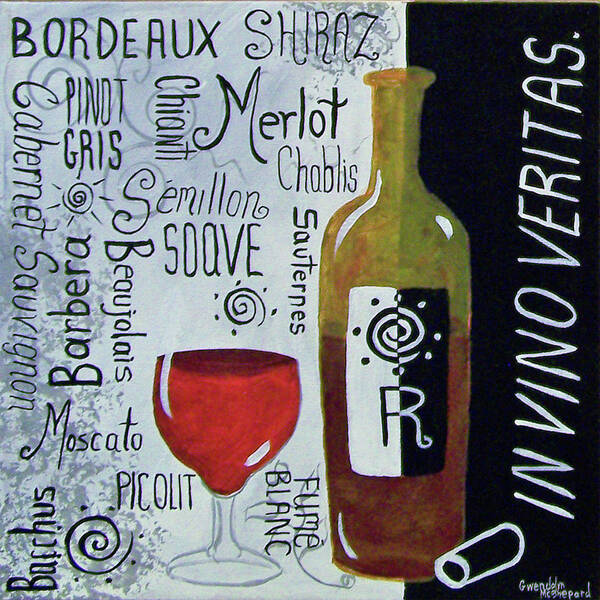This is a detailed painting of a wine bottle and glass. The wine bottle, depicted with green and reddish hues, features a distinctive label split between black and white halves. At the center of the label is a capital 'R,' with its left half being black on the white background and its right half white on the black background. Above the 'R' is a complex swirl design that also alternates colors, integrating into the label's domino-like design. The bottle is complemented by a wine glass filled with red wine to its left. 

The background of the painting plays with contrast and typography; the left two-thirds are white, while the right third is black. The black side prominently features the Latin phrase "In Vino Veritas," written vertically. Surrounding the bottle and glass, particularly on the white side, are names of various types of wine such as Merlot, Chablis, Bordeaux, Pinot Gris, Chianti, Moscato, and Sauternes. These names are creatively arranged in different fonts, sizes, and orientations, adding to the vibrant and eclectic visual texture of the artwork.

Additionally, there is a white outline of a wine cork to the right of the bottle, and at the bottom right corner of the painting, the artist's name, Gwendolyn McShepherd, is handwritten, providing a final touch of personal flair to the piece.